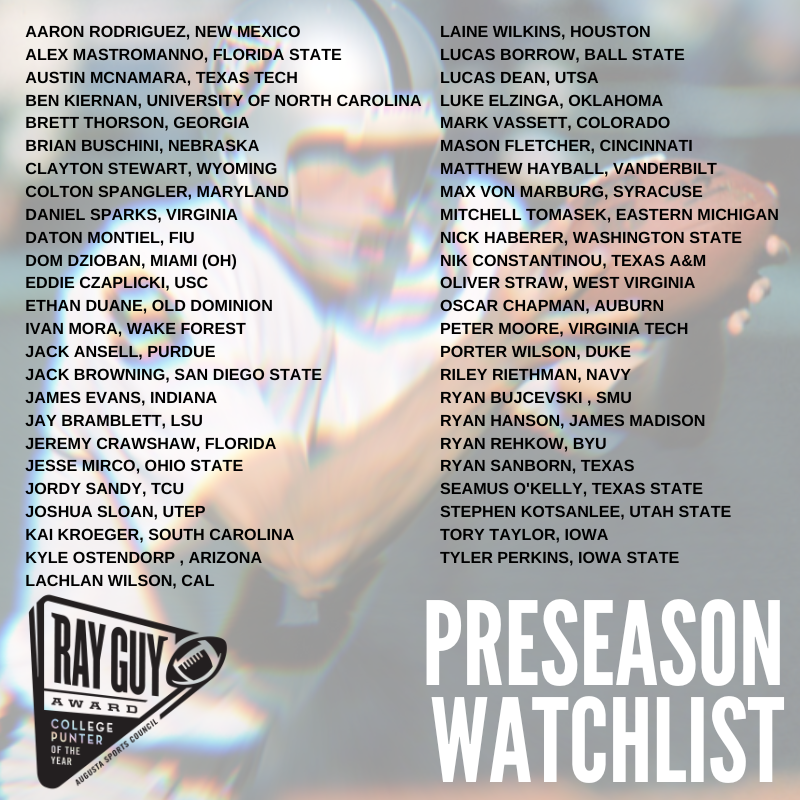The image is a detailed flyer for the "Preseason Watchlist" of the Ray Guy Award, which honors the College Punter of the Year. The flyer predominantly lists the names of punters and the universities they represent in alphabetical order from A to T. The names are displayed in black font, and include Aaron Rodriguez from New Mexico, Alex Mastromano from Florida State, Austin McNamara from Texas Tech, Ben Kiernan from the University of North Carolina, and many more. The background features a blurred image of a football player, who cannot be clearly identified, holding a football. In the bottom right corner, the words "Preseason Watchlist" are distinctly written in large white font. The bottom left corner contains a two-toned (white and black) triangular logo with a football at the top edge, denoted with the text "Ray Guy Award College Punter of the Year." At the top of the flyer, there is an image of Ray Guy in his Raiders uniform, ready to kick a football. This comprehensive list highlights the top contenders for the prestigious award, bringing attention to the college football punters to watch in the upcoming season.